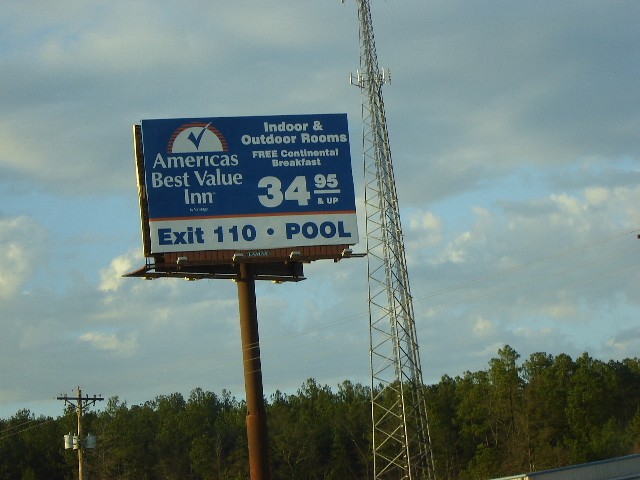This image showcases a billboard from a slightly upward angle, making the pole supporting the billboard, which appears to be a brownish color, quite prominent. Positioned next to the billboard, slightly to the right of the center, is a tall, slender cell tower that extends from the bottom to the top of the image. The photo seems to have been taken with the camera tilted slightly to the left, adding a dynamic perspective. In the background, a tree line is visible, with a clear sky stretching out above it. The billboard advertises "America's Best Value Inn" with a nightly rate of $34.95 and suggests taking exit 110 to reach the location.